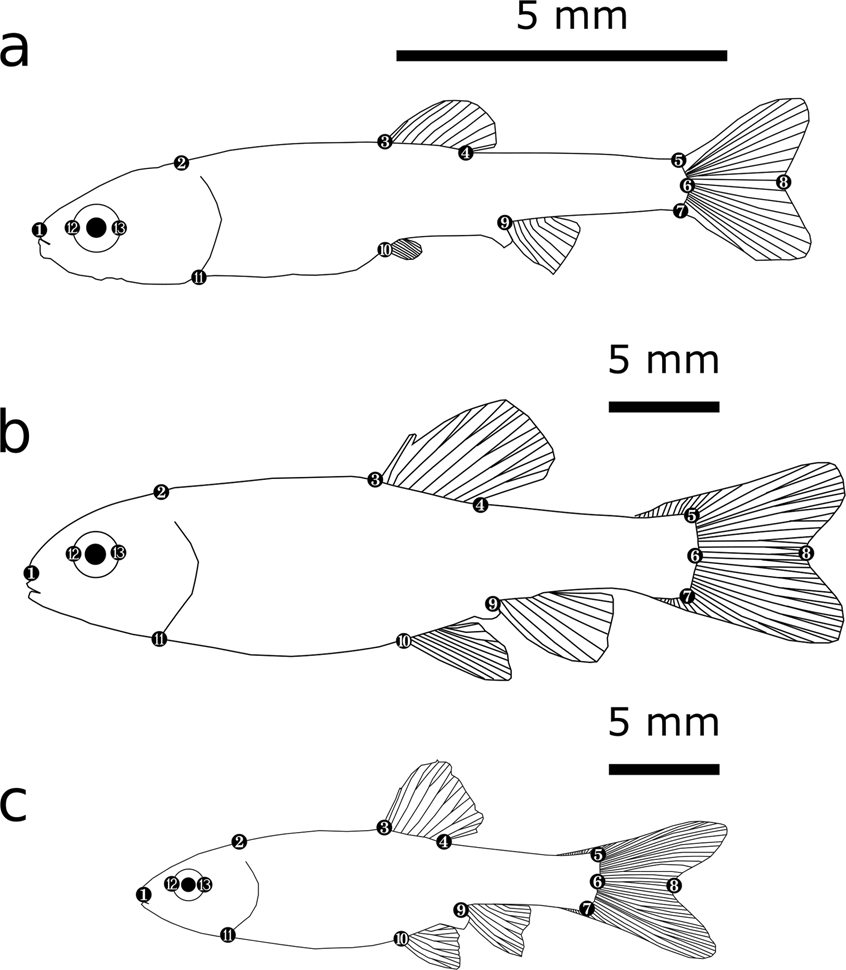This black and white illustration, likely sourced from a children's textbook or educational material, features three small fish displayed in a straightforward pen and ink style. Each fish is presented in profile and stacked vertically, labeled as A, B, and C from top to bottom. Above each fish, a black bar denotes a scale of 5 millimeters, emphasizing the small size of these aquatic creatures. The top fish, labeled A, appears almost entirely encompassed by the 5mm scale, highlighting its diminutive stature. Each fish is intricately annotated with numbers ranging from 1 to 13, marking specific parts of their anatomy such as the mouth, eyes, fins, and tail. While the illustration does not include a visible key, it suggests the presence of a legend elsewhere, likely explaining the significance of each numbered label. The bottom fish, resembling a guppy in shape, underlines the diversity among these small specimens. Overall, the drawing serves as a detailed anatomical guide, meticulously labeling each section of the fish for educational purposes.